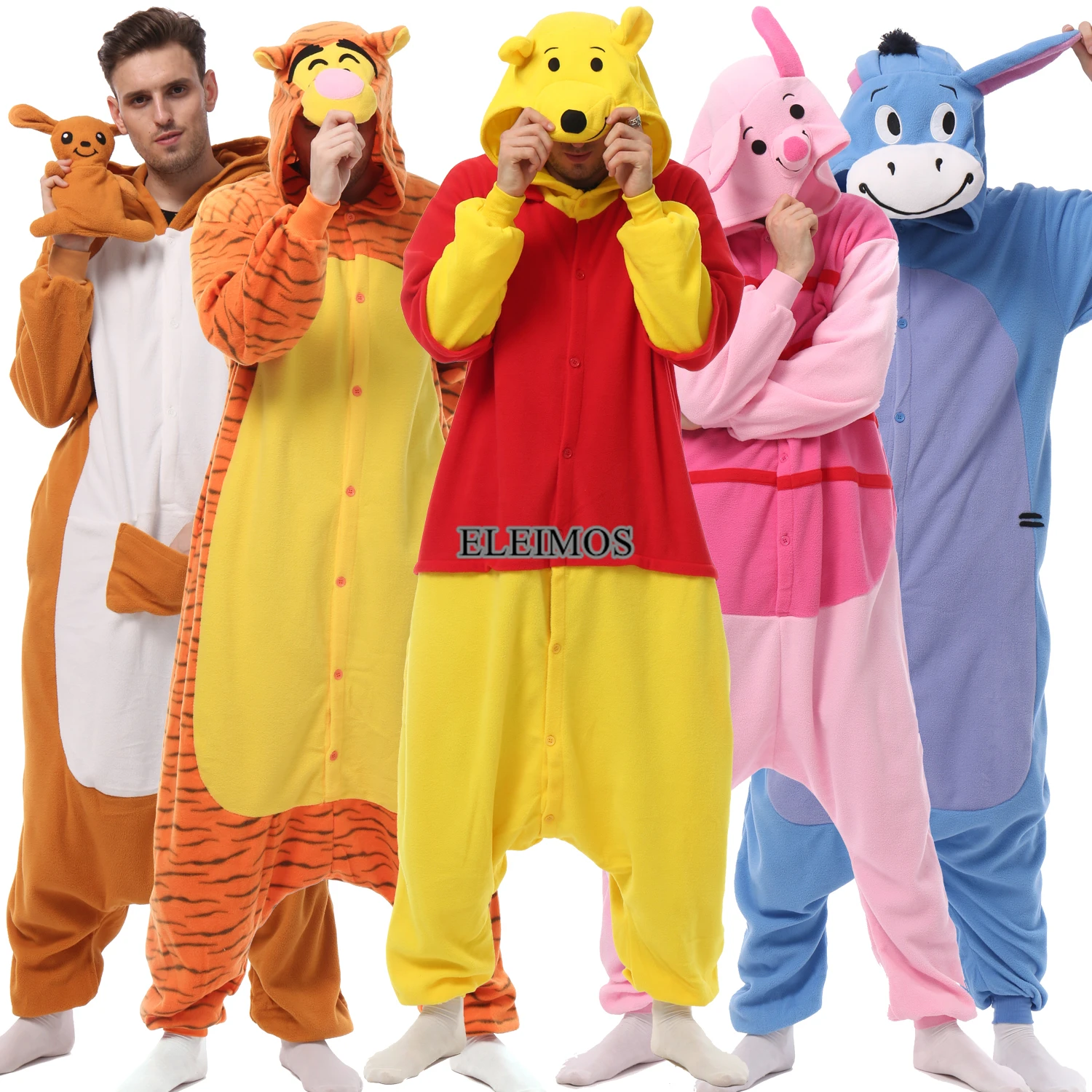The image is a realistic, stock photo showcasing five adults dressed in vibrant, oversized onesies inspired by Winnie the Pooh characters, set against a plain white background. From left to right: the first person is a white male in his 20s or 30s with black hair, wearing a kangaroo onesie without the hood on, revealing his face, and holding a small kangaroo doll. Next to him is someone in a colorful Tigger costume, complete with orange and black stripes and a yellow belly, holding the character hood over their face. The central figure wears a red and yellow Winnie the Pooh onesie with the hood completely covering their head. To the right of Pooh is a person in a pink Piglet onesie, also holding the hood over their head in a thoughtful pose. Finally, the far-right figure is in a blue Eeyore onesie, lifting one of Eeyore's ears with the hood obscuring their face. All are standing in white socks and the text "Elimos" appears centrally on the image as a possible brand watermark.